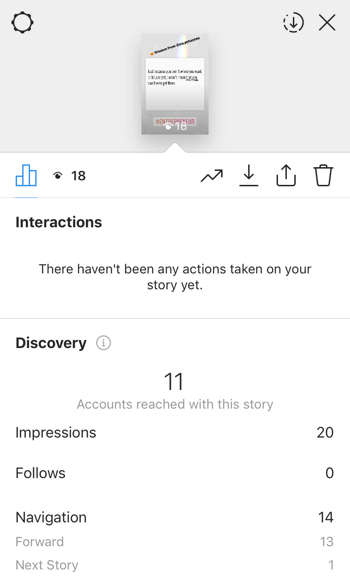A detailed and properly formatted caption for the described image could be:

---

This image appears to be a screenshot showcasing the insights and statistics of an Instagram story post. At the top of the screenshot, a minimized version of the original story post is displayed, making it difficult to read the specific content. The image reveals that the story has received a total of 18 views.

Below the post preview, the insights are divided into several sections. The first section is labeled "Interactions," which reports that there have been no actions taken on the story yet.

On the left side of the insights, the section is titled "Discovery." Here, it is noted that the story has reached 11 accounts and accumulated 20 impressions. Additionally, the statistics under "Navigation" indicate that there have been 14 navigation actions: 13 forwards to the next content and 1 instance of navigating to the next story.

Lastly, the text color within the different sections varies, with most of the letters in black and the final two sections, likely indicating "Navigation" details, appearing in gray.

---

This caption provides a comprehensive description of the image, detailing each section and the numerical insights present in the screenshot.